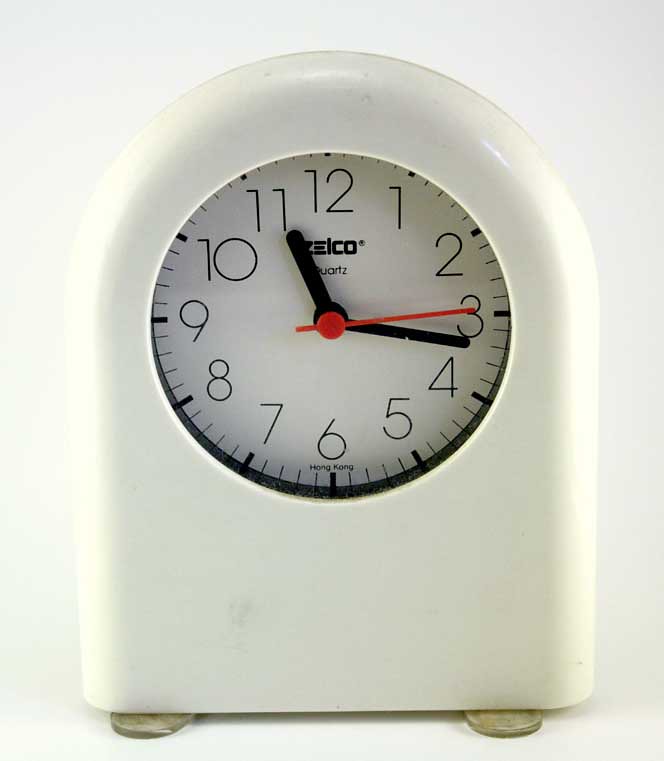This detailed indoor color photograph showcases a small, slightly used plastic clock, perfect for a nightstand. The clock, which stands about 8 inches tall and 3 to 4 inches wide, has a distinctive shape, with a rounded top and a squared-off bottom. It's supported by two semi-transparent feet located at the bottom corners. 

The clock's face is off-white, with black numerals in a traditional arrangement from 1 to 12. The hour and minute hands are black, while the second hand is red. The time displayed is 11:17, with the second hand pointing at the 3. Just below the 12 o'clock position, the brand name "ZELCO" is printed, followed by the word "quartz," although the initial "Q" is obscured by the hour hand. Additionally, below the 6 o'clock position, the words "Hong Kong" are visible in black letters. The clock's plastic surface exhibits slight signs of wear, giving it a somewhat dingy appearance.